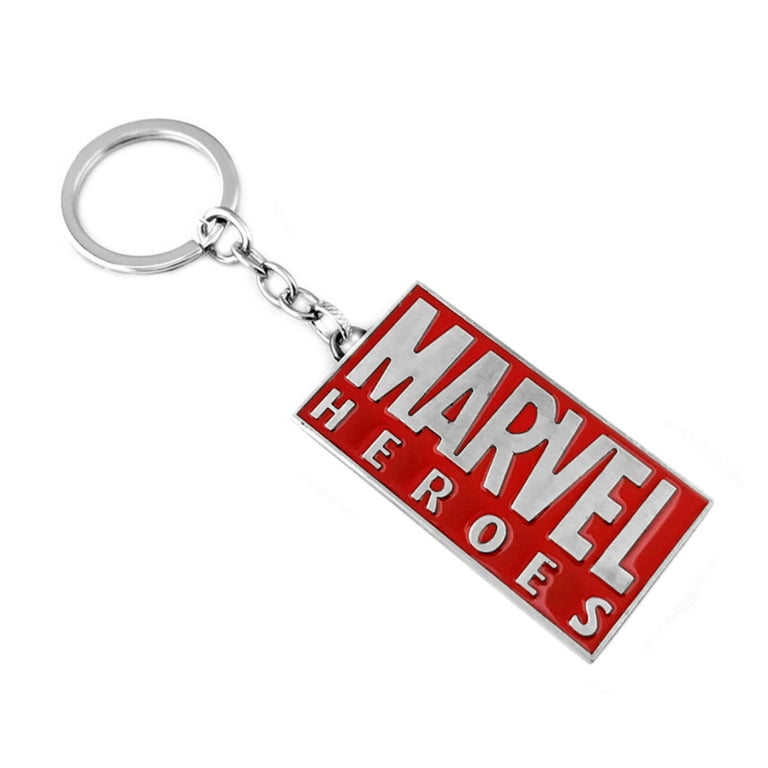The image features a high-quality, close-up photograph of a keychain displayed on a white background, making it appear geared towards online sales. The keychain comprises a bright silver metal ring attached to a short, five-link chain, which leads to a rectangular emblem diagonally positioned from the upper left to the lower right. The emblem itself is a vivid red rectangle with a silver border. In its center, "MARVEL" is prominently etched in large, classic Marvel font, while "HEROES" is written below in equally capitalized but smaller, spaced-out silver letters. The visible portions of the keychain exhibit a sleek and polished finish, indicating a well-crafted product.